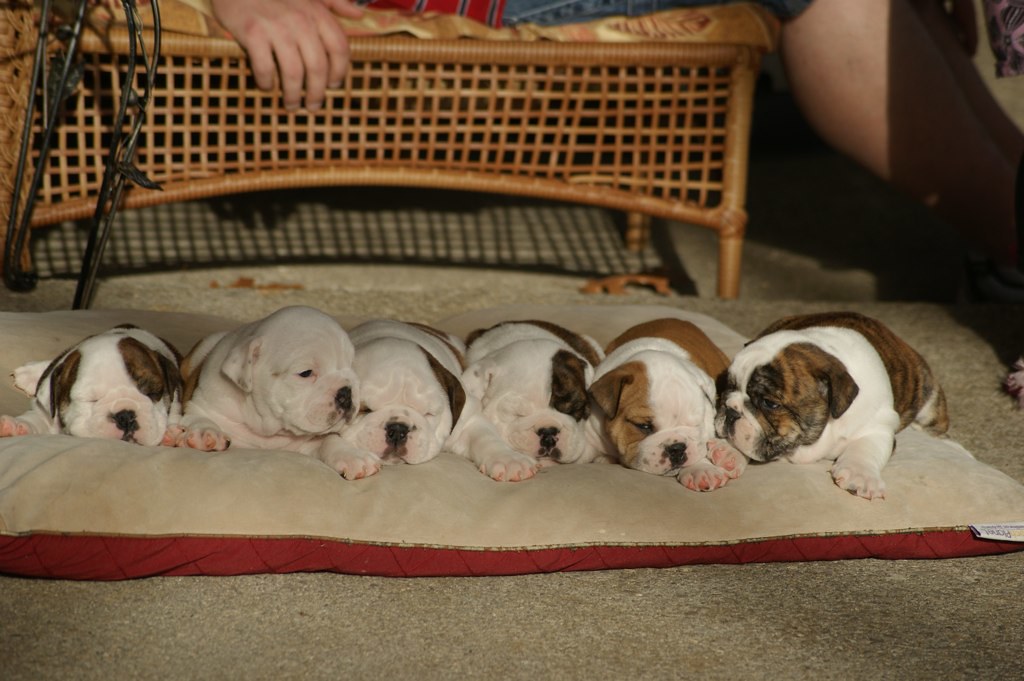This digital indoor photo captures six adorable English Bulldog puppies, uniformly distributed on a large beige and red blanket placed over a cream-colored rug. The puppies, each exhibiting distinct patterns of white and brown patches, are all facing the camera with most of them appearing to be asleep or lazy, with their endearing, wrinkly foreheads and snouts slightly relaxed. The first puppy on the left is predominantly white with brown spots around its ears and eyes. The second puppy is entirely white, the third one shares this white coat except for a brown patch on its right ear. The chubby fourth puppy has brown markings over its right eye, ear, and near the rear. The fifth, lighter-brown puppy has coloration on its left eye, ear, and mid-back. The sixth and final puppy on the far right has a mix of brown spots on its right eye, ear, around its mouth, and extending down its back. In the background, there's a tan wicker chair with a weaved design, partially obscured by a Caucasian hand resting atop it. Sunlight streams from the bottom right of the image, adding a warm glow to the serene scene.